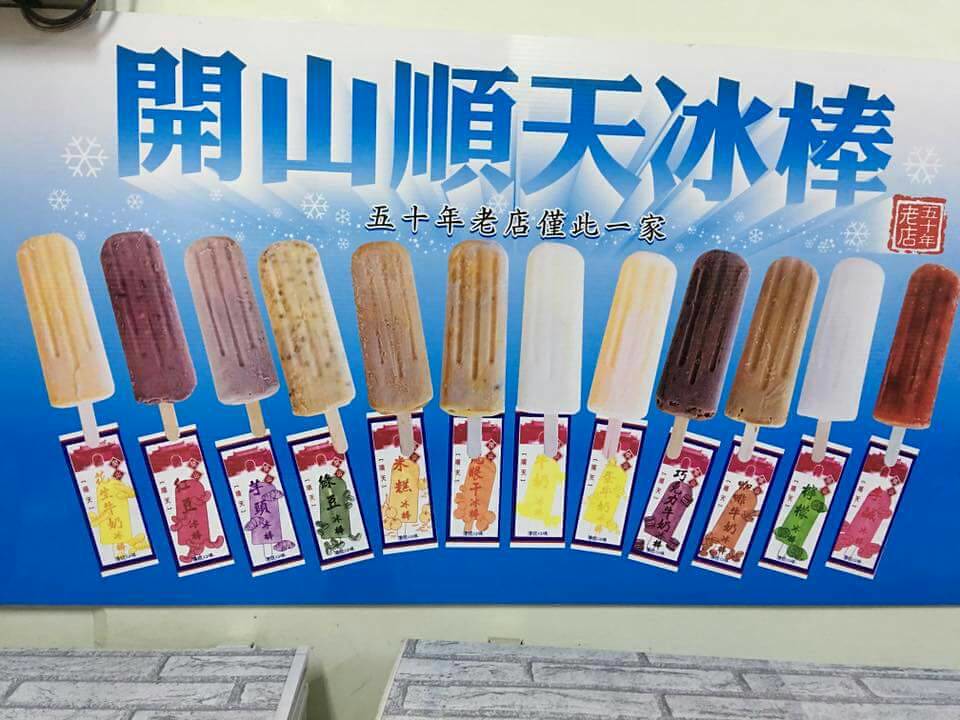A detailed color photograph capturing an advertisement poster on a light yellow wall. This vertically oriented poster features a gradient background, transitioning from white at the top to dark blue at the bottom, adorned with delicate snowflakes. At the very top center, large blue characters in an Asian language create a dramatic effect, fanning outwards and surrounded by a vibrant aura. Just below, additional Asian text in a smaller black font with a large white border adds informational context.

The focal point of the poster showcases 12 distinct popsicles, each mounted on a single stick, arranged in a slight arch from left to right. These fruit bars span a spectrum of pastel shades, including soft tans, browns, purples, pinks, yellows, whites, and cream colors. Each popsicle has a corresponding rectangular vertical label beneath its stick, featuring text in an Asian language.

The presence of faux brick-lined shelves at the bottom of the image adds a contrasting texture to the scene, enhancing the lively and appetizing display of the popsicles. The combination of the colored popsicles against the gradient background with the textual elements creates an eye-catching and detailed advertisement.